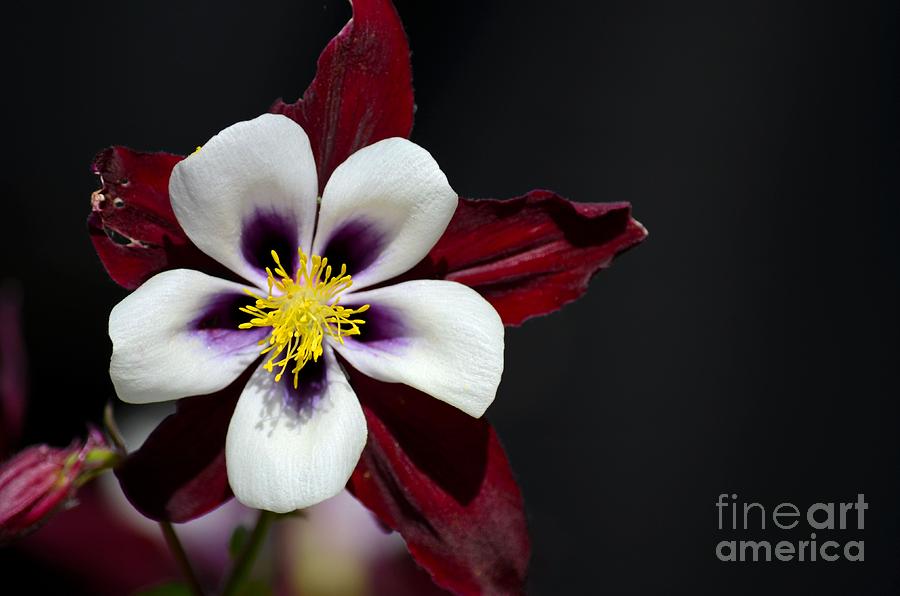This close-up photograph captures a stunning flower with vibrant details. The flower features five large, starfish-like red petals that form the outer layer. In front of these are five rounded white petals adorned with delicate purple blotches at their center. The heart of the flower bursts with vibrant yellow tendrils, creating a striking contrast against the surrounding colors. Adjacent to the main flower, a pinkish-red bud remains partially closed, adding depth to the composition. The background is artistically blurred in a dark, bokeh style, enhancing the flower's vividness. This photorealistic image includes the watermark "Fine Art America" in white text at the bottom right corner.